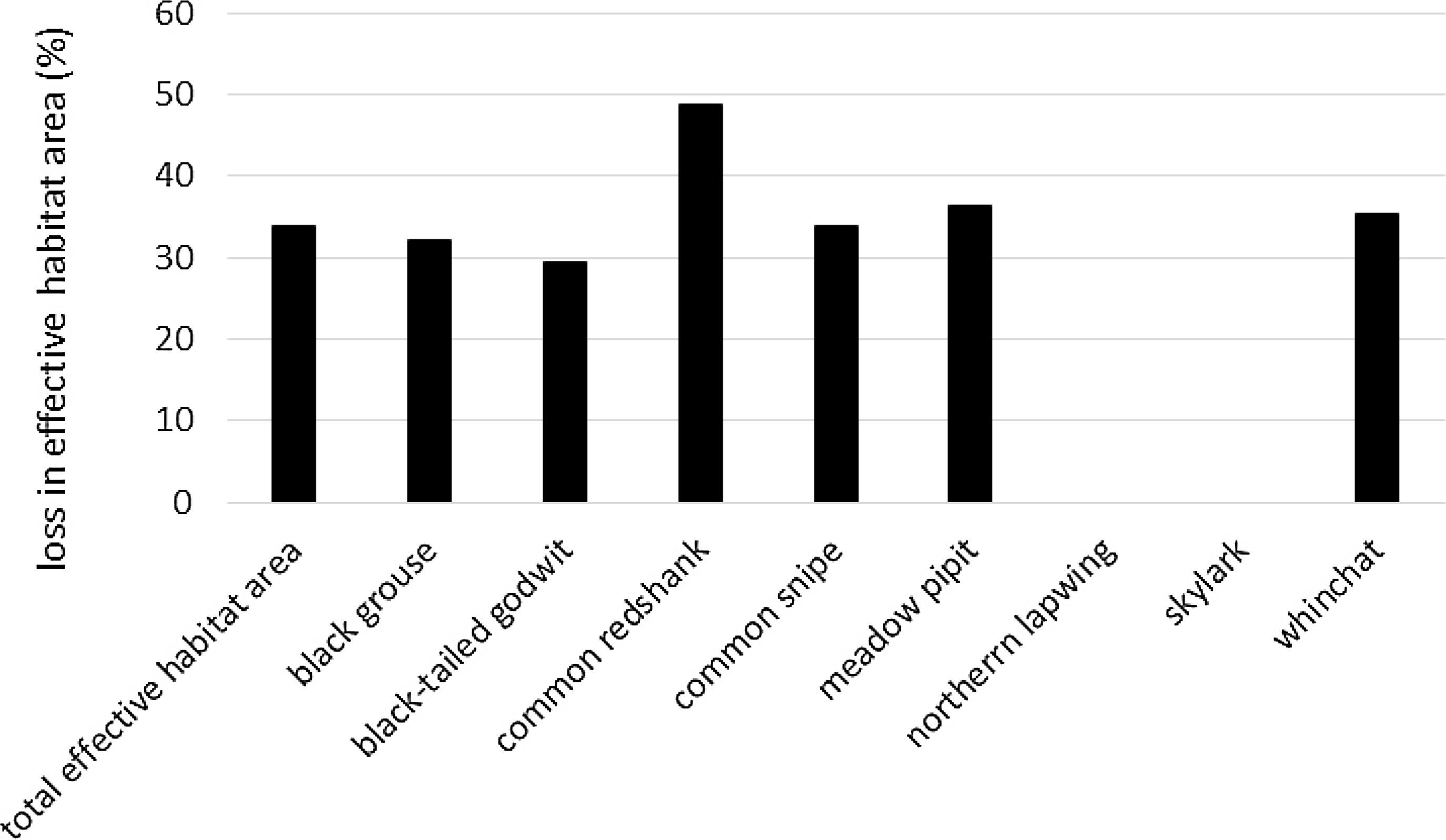The image depicts a bar chart illustrating the loss in effective habitat area (%) for various bird species. On the y-axis, labeled "Loss in Effective Habitat Area (%)" in black font, the values range from 0 to 60 in 10-unit increments. On the x-axis, under the overarching label "Total Effective Habitat Area," are the names of several bird species enumerated diagonally: Black Grouse, Black-tailed Godwit, Common Redshank, Common Snipe, Meadow Pipit, Northern Lapwing, Skylark, and Whinchat. The bars on the chart vary in height, with most of them centered around the 30% mark—Black-tailed Godwit being the lowest at approximately 30%, while Common Redshank stands out with a significantly higher loss of around 47%. Notably, the Northern Lapwing and Skylark do not have any bars, indicating no recorded loss for these species. The chart also features light gray grid lines across the background to help gauge the percentage values more precisely.